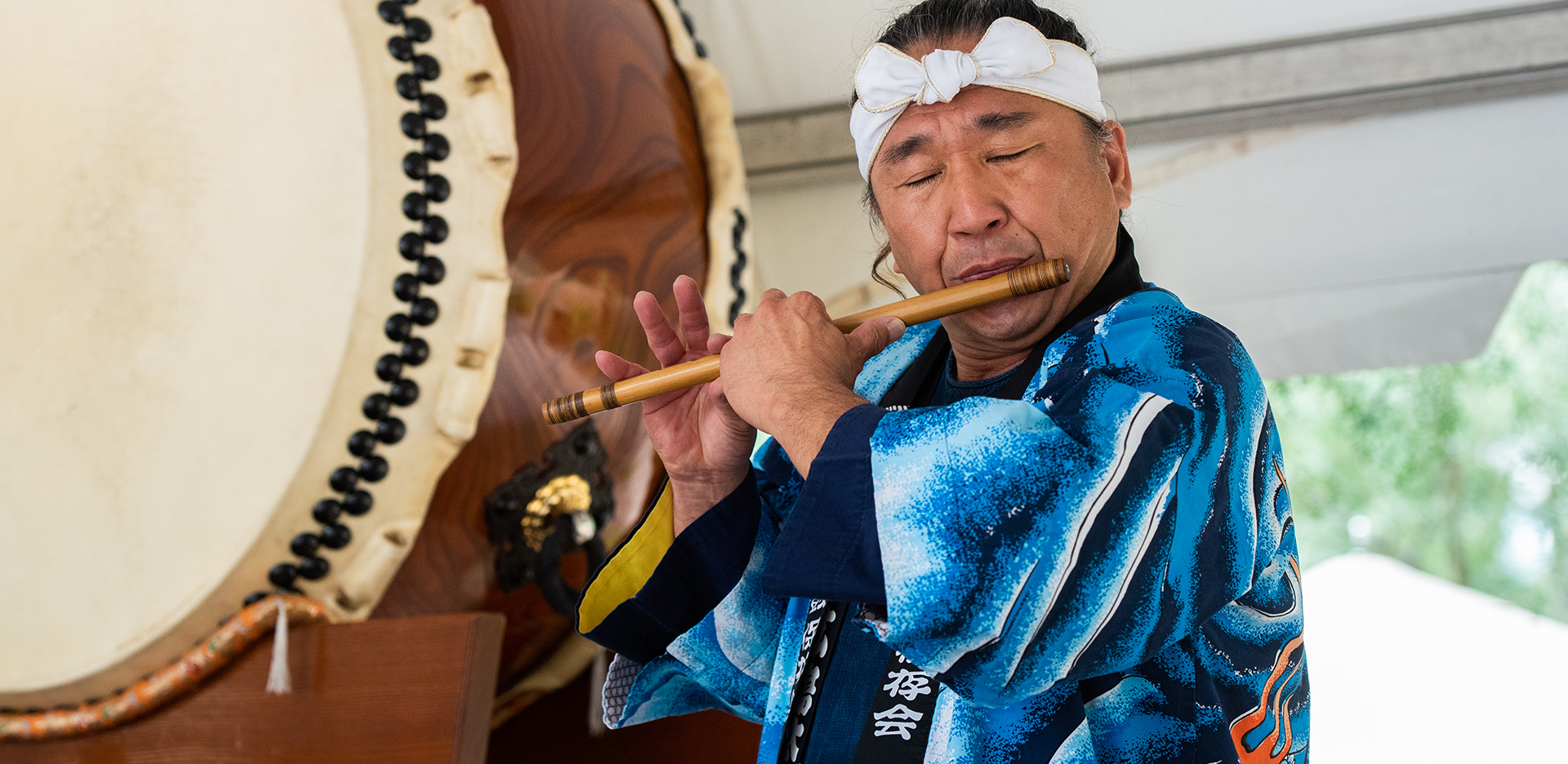In the horizontal image, a man is shown playing a wooden flute with his eyes closed. He is an older man with short black hair, wearing a white headband tied in a bow at the front. His outfit is a striking blue kimono featuring various shades of blue and some white accents, along with a visible red design on his back and hints of yellow material inside the cuff. The collar of the kimono displays what appears to be Japanese writing. To the left of the man, there is a large, beige and brown Taiko drum laid on its side and resting on a stand adorned with cushions and white tassels. The background features a hint of outdoor light and greenery, suggesting an indoor area with a white roof and a gray ceiling in the upper right corner.